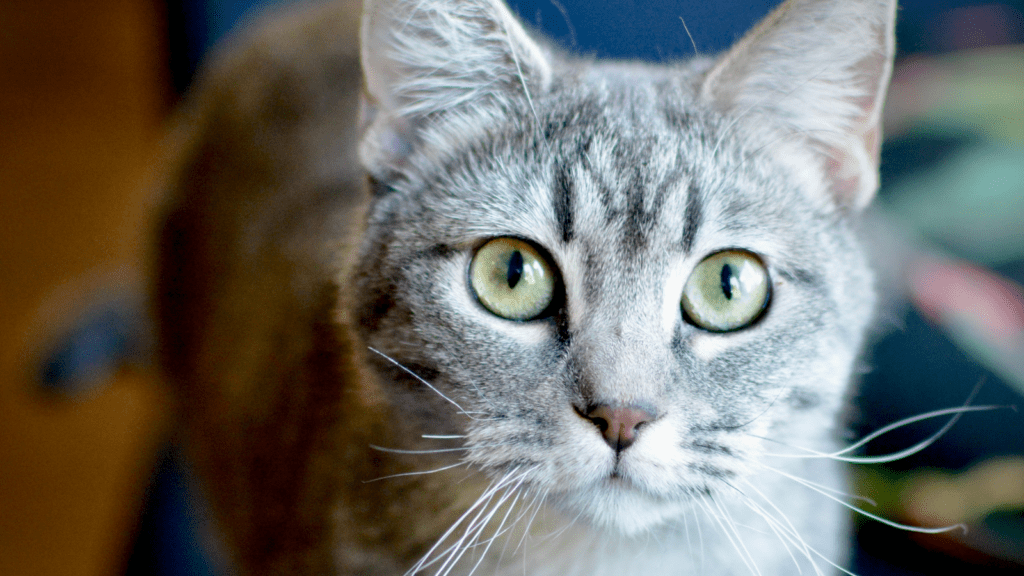This is a close-up photograph of a house cat with its face prominently in focus, looking directly at the camera with an inquisitive expression. The background, blurred and unfocused, features a mix of blue, brown, yellow, pink, and green hues, and the cat's back body is also softly obscured. The cat's fur is a mix of gray and white, with darker black lines creating a distinctive pattern, including an 'M' shape on its forehead. The cat's face, crisply detailed, showcases light green eyes lined in black and a cute little pink nose. The cat's ears stand up with their pink inner coloring visible, and white whiskers fan out in every direction. Additionally, the cat's chin and part of its upper body are white. The overall appearance of the cat is gray with hints of brown tones near the face due to the lighting.